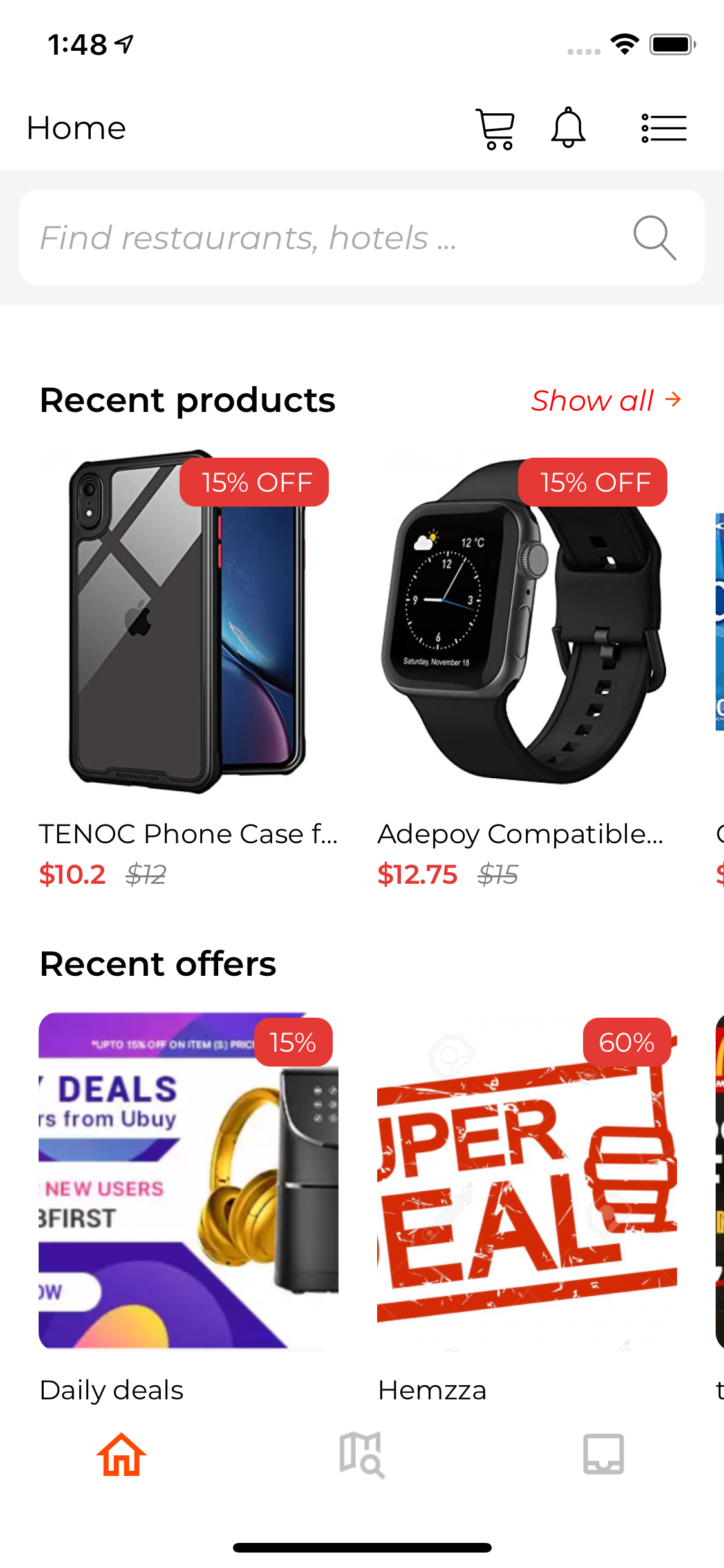This screenshot depicts the home screen of a shopping app captured at 1:48, with the device showing a full battery. Prominently featured at the top of the screen is a search bar with the placeholder text "Find restaurants, hotels." To the right of the search bar are three icons: a shopping cart, a bell for notifications, and a menu for additional options.

Below the search bar, the app displays recent products on sale, including a Tenok phone case priced at $10.20, currently offered at a 15% discount. Adjacent to it is an Adapay-compatible smartwatch, also discounted by 15%, bringing its price to $12.75.

Further down, the app highlights recent offers. This section features "Daily Deals," which are uniformly marked down by 15%, and an item called "Hamza," impressively discounted by 60%.

The navigation bar at the bottom of the screen includes three main icons: an orange home icon on the bottom left for returning to the home screen, a map with a magnifying glass in the center for location-based searches, and an inbox icon on the bottom right for accessing messages.